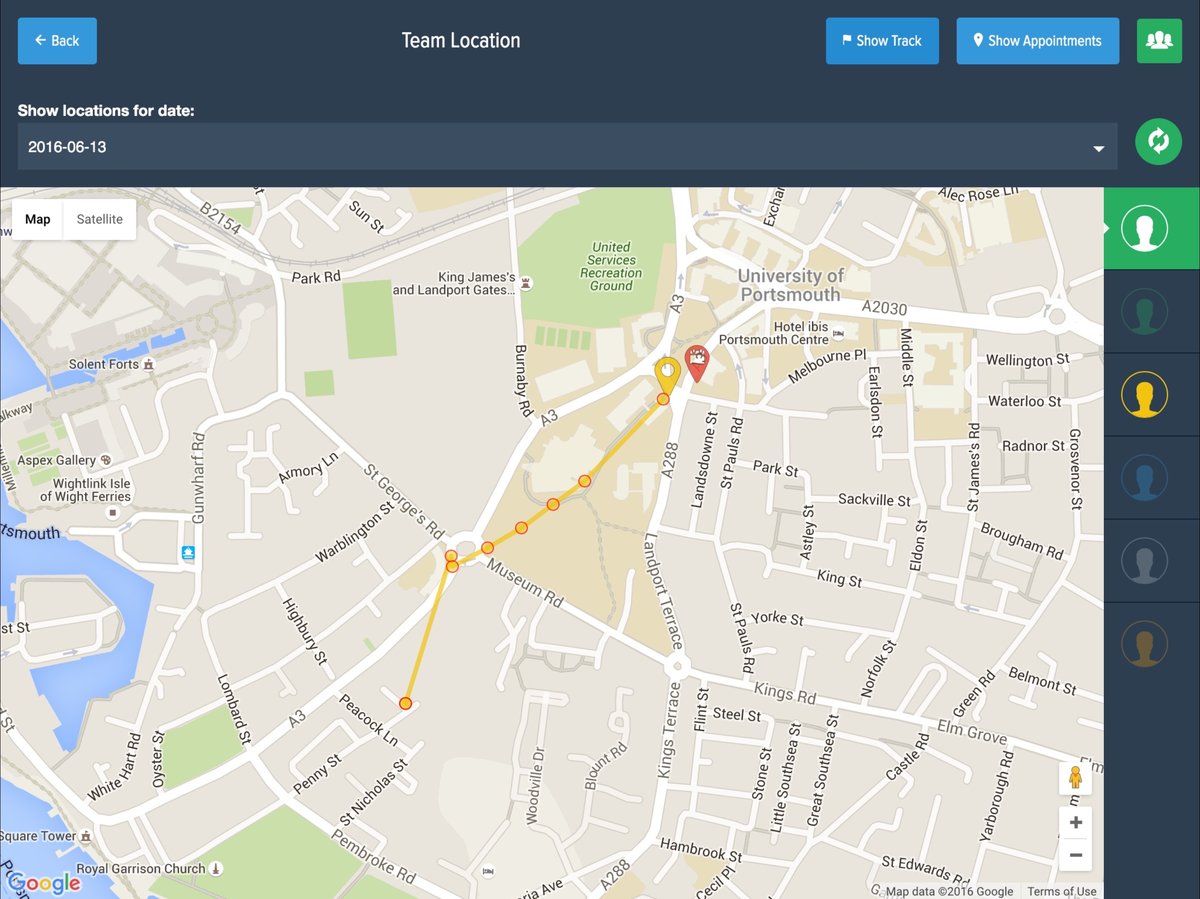This image is a screenshot from a website displaying team locations. In the upper left-hand corner, there's a prominent blue back button. The top center features the title "Team Location" in white font against a blue background. In the upper right-hand corner, three buttons are visible: the first is an icon displaying three people, the second is labeled "Show Appointments," and the third is labeled "Show Track."

Beneath the title, there is a section for entering a date labeled "Show Location for Date," with an input bar directly below it. The date "2016-06-13" has been entered in this bar. Adjacent to the input bar, a green circular refresh button is prominently displayed.

On the right-hand side of the screen, there are six head icons, each in a distinct color. The top icon, highlighted in green with a white person icon, is currently selected. The subsequent icons are colored green, yellow, blue, gray, and orange respectively.

At the center of the screen, the layout features a city map that outlines the streets but does not display individual buildings. An orange line, indicating a specific route taken, is visible on the map, extending to an orange pin that marks the end destination. Along this orange route, there are eight circular stop points indicating key locations or events.